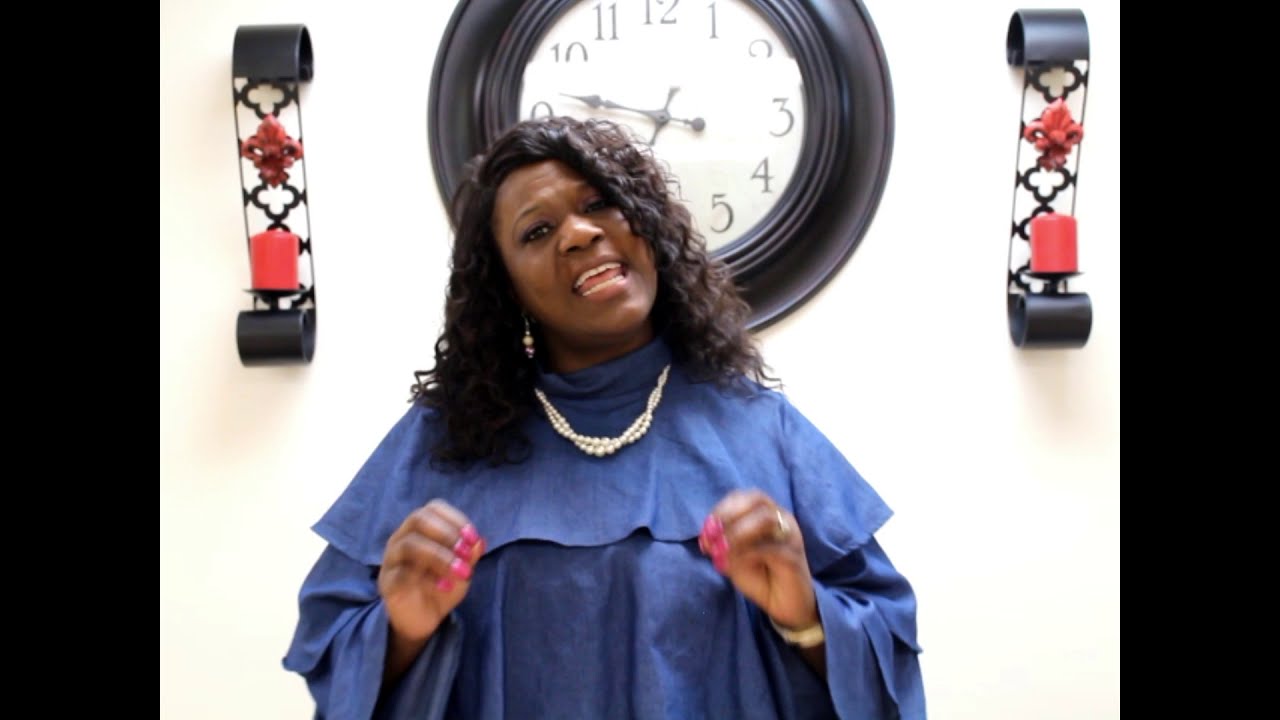The image depicts an African-American woman standing and facing forward with her head tilted to the left, appearing to sing or speak. She has curly black hair that extends just past her shoulders, and her mouth is open, revealing both her top and bottom rows of teeth along with her tongue. She is dressed in a dark blue gown with an overlay top that drapes down to her wrists. The outfit resembles a robe. Around her neck, she wears two intertwined pearl necklaces, and she has a gold watch on her right wrist and pink fingernail polish on both hands. Her hands are positioned near her chest. Behind her is a white wall with a slightly yellow shade, featuring an analog clock with a light reflection near the number 10. The clock has black hands indicating approximately 9:35. Flanking the clock are two identical wall decorations that resemble stylized fleur-de-lis designs, holding pink candles at the bottom.